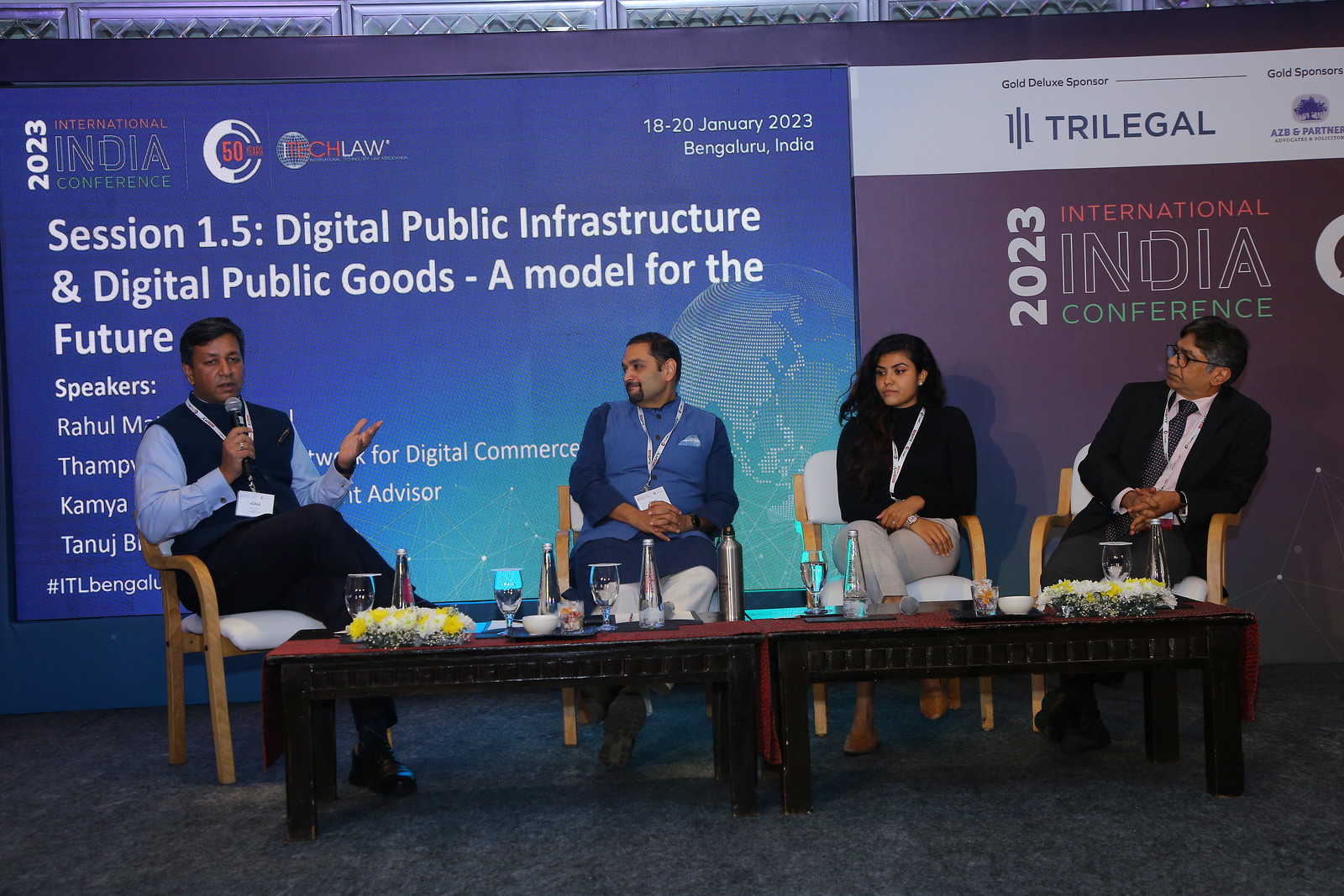This photograph captures a panel discussion at the 2023 International India Conference, held from January 18 to 20 in Bhargava Fero, India. The backdrop prominently features multiple displays with information about the conference, including a logo and the text "Trilegal 2023 International India Conference." The setting is indoors, carpeted in gray, and the participants are seated on wooden chairs with gray cushions around two low wooden tables. The tables hold bottles, glasses of water, bowls, and two bouquets of flowers.

Four people are engaged in this discussion. On the far left, a man in a black vest over a blue long-sleeve shirt and black pants speaks into a microphone, his arm extended. Next to him sits another male panelist wearing a blue multicolored shirt and khaki pants. To his right is a woman with black hair dressed in a black shirt and khaki pants, accessorized with a wristwatch. The final participant on the far right is a man in a black suit with a black tie and a white shirt. All participants are wearing lanyards.

Behind the speakers, there are LED screens displaying various session details. Notably, one screen reads "Session 1.5: Digital Public Infrastructure and Digital Public Goods – A Model for the Future," listing speakers Rahal M and Tanuj B, among others. There’s also a visible watermark on the top right-hand corner of the slide that states the conference dates and location: "18 to 20 January 2023 Bengaluru, India," along with the Tech Law logo featuring the number 50 inside a globe.